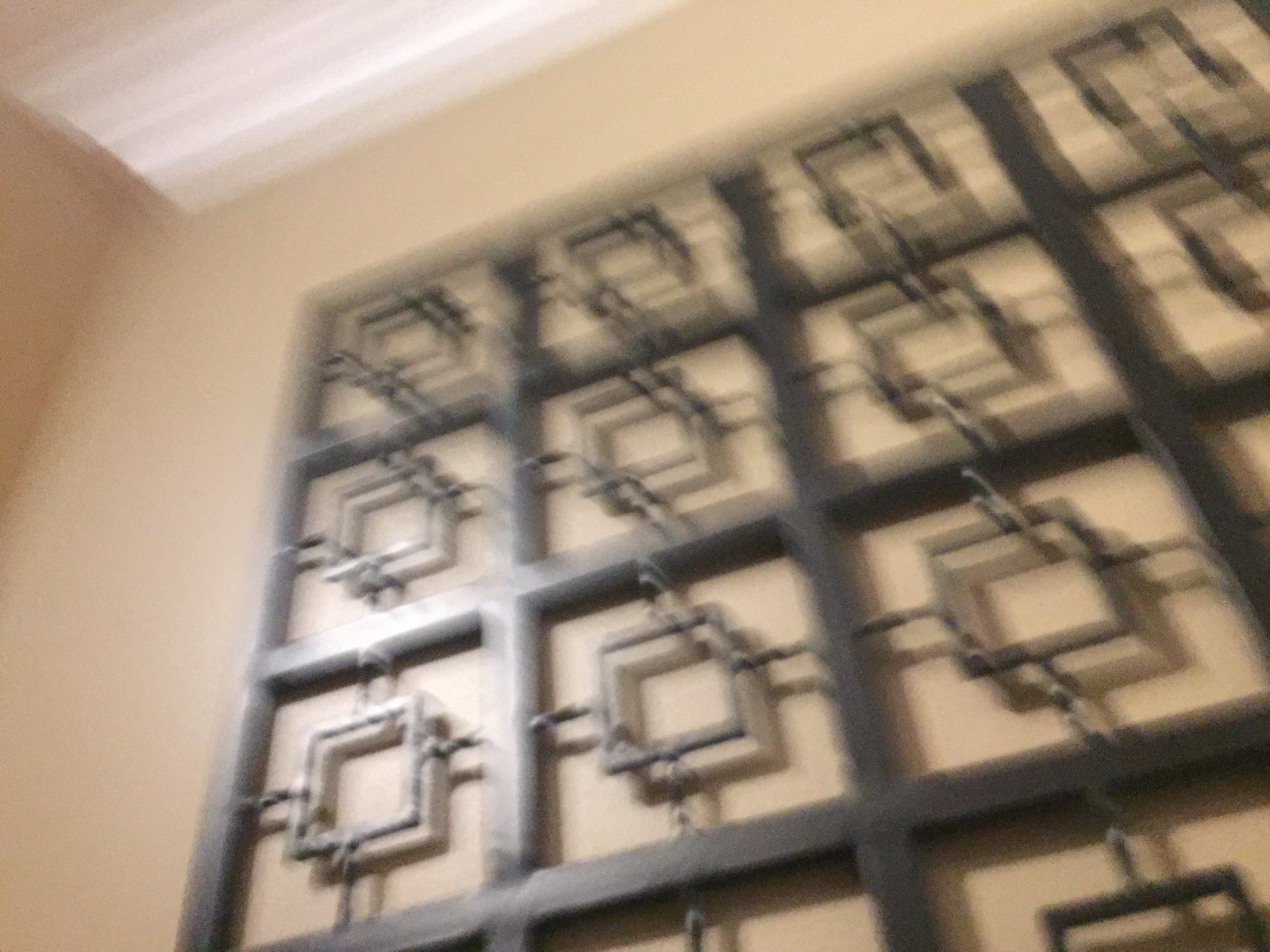The image is a blurry, out-of-focus photograph of a room with beige-colored walls and a white ceiling. The centerpiece of the image is a decorative wall hanging designed in a square grid pattern. The hanging, which appears to be made of dark, possibly metal material, is comprised of numerous smaller squares forming a larger square. Each smaller square houses an additional metal square suspended by hooks or chain links, creating a layered, overlapping effect. The structure gives an artistic, contemporary feel to the space, adding texture and visual interest against the plain wall.